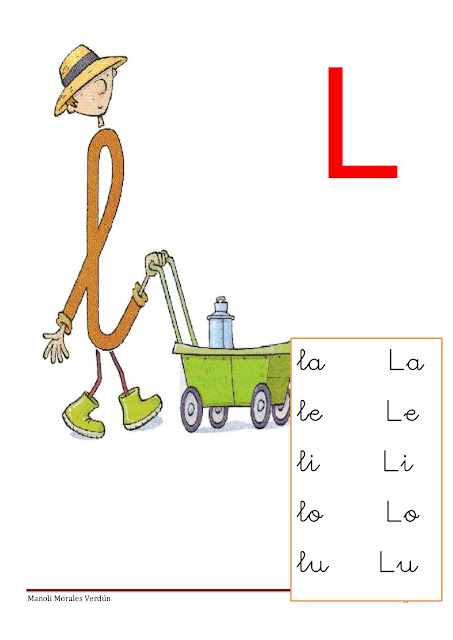The illustration appears to be a vibrant and whimsical scene from a children's spelling book, specifically designed to teach cursive writing. Dominating the image is a playful character whose body is cleverly shaped like a cursive L. This character is a man adorned in an orange shirt with yellow sleeves, a wicker hat with a black band, and green shoes. He is seen pushing a small green cart, which resembles a wheelbarrow, complete with a water bottle inside.

To the right of this character, a large red letter L in block form stands out prominently. Below, a rectangular text box provides a detailed lesson on the letter L in both cursive and regular fonts. This box showcases the various ways to pair the letter L with different vowels, displaying combinations such as LA, LE, LI, LO, and LU. Each pair is represented in cursive on the left and regular block lettering on the right, emphasizing the transition between the two styles for educational purposes.

Overall, this scene is a fun and engaging educational tool designed to help young children learn the different ways to write and use the letter L in cursive, while also enjoying the delightful cartoon-like illustration of the man with the noodle-like, cursive L body.